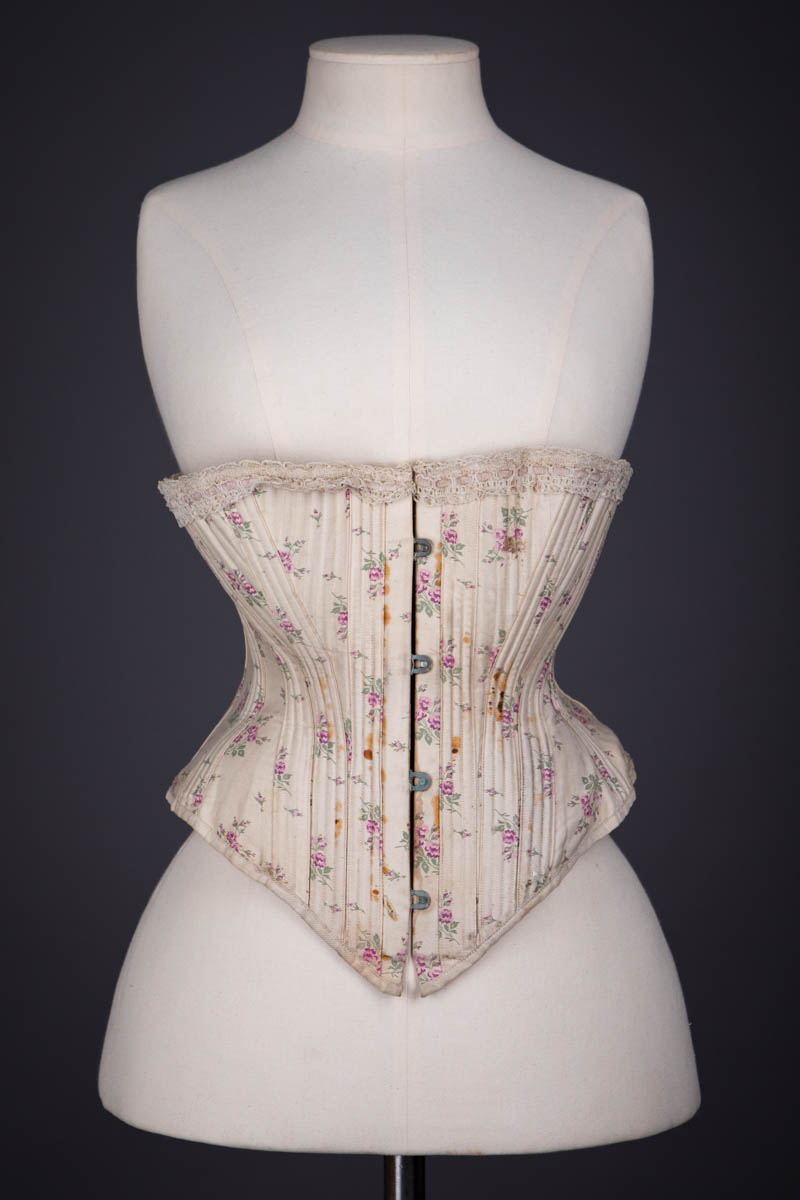Against a black background, the image features a white mannequin displayed from just below the neck to the hips, emphasizing its feminine curves. The mannequin is adorned with a predominantly white corset, which accentuates the waist to create an hourglass figure. The corset extends from slightly below the chest area down to the hips, forming a V shape at its lower edge. It is embellished with delicate lace around the top and is decorated with clusters of pink roses interspersed with green leaves throughout the fabric. The corset fastens at the front with hooks connected to bobbin-like mechanisms, enhancing its form-fitting design.